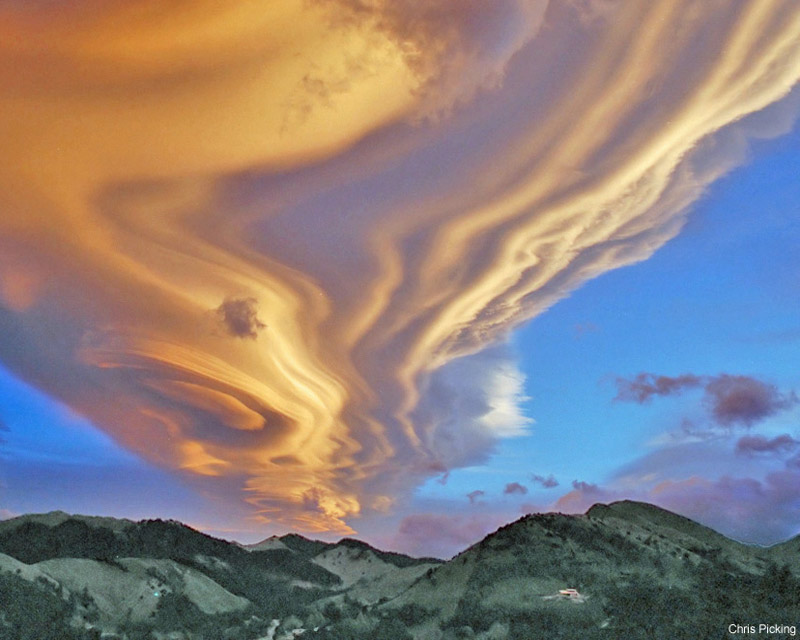This image captures a mesmerizing painting or colored drawing of a dynamic landscape where the sky takes center stage. At the top, ominous and peculiar-looking clouds dominate, stretching from the upper left corner to the middle, then cascading down toward the center in streaky yellow and gray lines. The clouds on the right, light-colored with ripples, descend from the upper right corner, converging with those on the left just above the horizon, creating a meeting point slightly left of center. Below this turbulent sky are lush, green hillsides, dotted with dense forests, extending across the left, middle, and right of the image, with the hills on the right appearing closest to the viewer. The horizon just above these hills has a purplish hue, suggesting a setting or rising sun. A touch of blue sky peeks out from behind the ominous clouds on the upper right, enhancing the overall vividness. In the bottom right corner, the artist's signature, "Chris," is visible although the last name is unclear. The interplay of glowing blue, amber yellow, and purple hues in the sky, possibly created through a time-lapse technique, adds a majestic and almost surreal quality to the scene, as though the clouds are in constant, fluid motion.